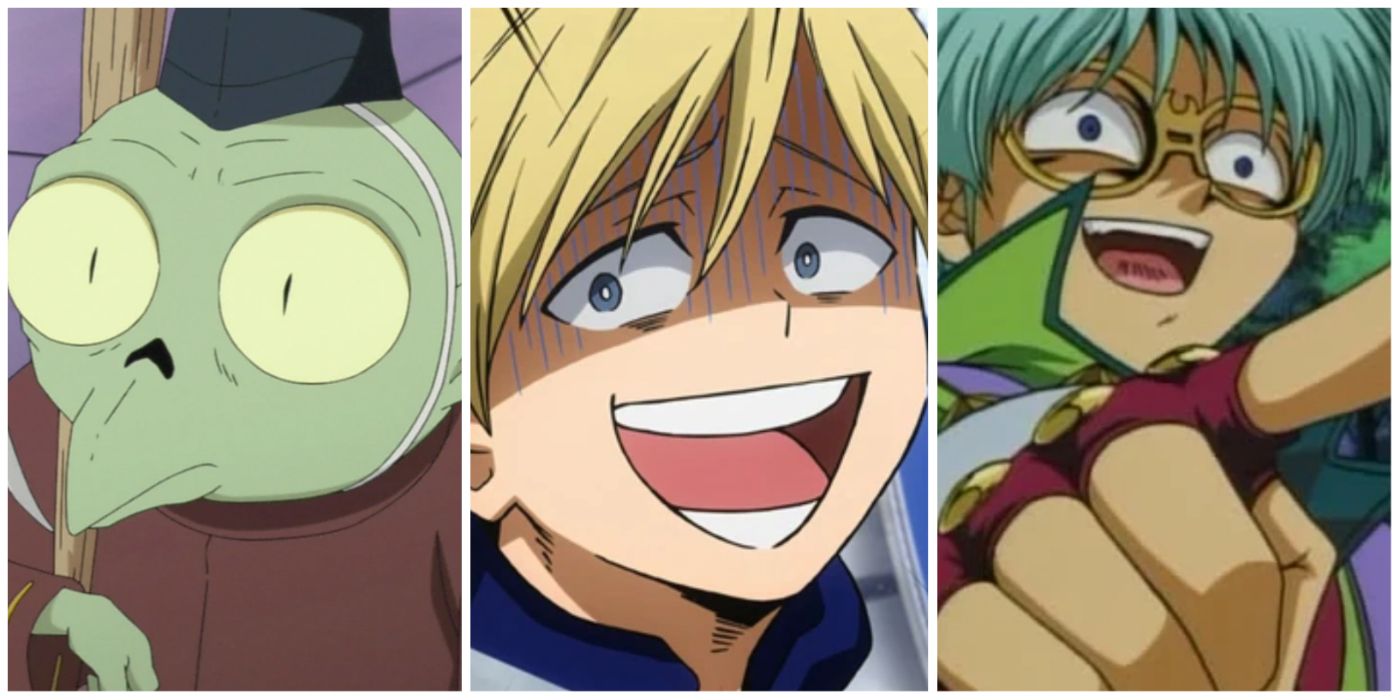The image is a collage featuring three distinct screenshots from different anime series. On the far right, there is a close-up of Weevil from Yu-Gi-Oh! He has green hair, wears glasses, and points to the right with a fingerless red glove. In the center, the character resembles Naito from My Hero Academia, with blonde, pointed hair and a cheerful expression. On the far left, there is Jaken from Inuyasha, a non-human character with green skin, bug-eyed features, and a beak-like mouth. The collage highlights the unique appearances and distinct traits of the characters from their respective anime.